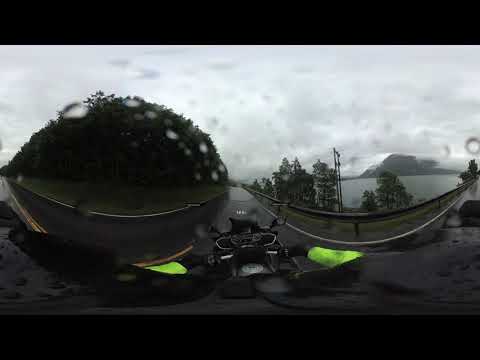The image captures a dramatic, first-person perspective from a rider on a motorcycle navigating a wet, winding road. Taken with a 360-degree view and featuring a fisheye lens effect, the scene is vividly rainy with visible raindrops on the camera lens. The rider is clad in a bright green jacket with black gloves, gripping the handlebars. The road ahead stretches forward, with a guardrail to the right and a significant slope leading down to a large body of water, surrounded by trees and greenery. On the left, the road forks, with one path continuing straight and the other veering left, both flanked by thick forested areas. The background showcases an overcast sky, dark and heavy with rain, with a mountain visible on the horizon, emphasizing the remote and adventurous setting. The black borders at the top and bottom of the image frame this thrilling ride scene perfectly.